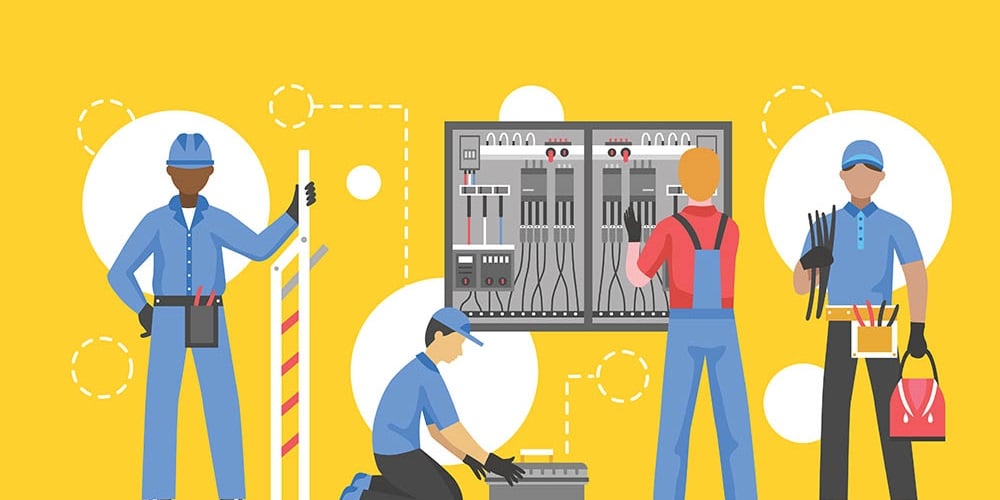This image is a cartoon-style drawing of four men engaged in various construction and electrical tasks, set against a predominantly yellow and white background. The men appear to be electricians or handymen, working diligently in different positions. On the left, an African-American man with a hard hat is gripping a ladder, contributing to the electrical setup. Next to him, a man kneels on the ground, wearing gloves and operating a toolbox. To his right, another man, faced away from the viewer, is focused on adjusting an electrical box. Finally, on the far right, a man stands with a tool belt around his waist, holding a bundle of wires in one hand and a red bag in the other. Although the men are depicted without facial features, the detailed use of colors such as orangish yellow, blue, lighter blue, beige, orange, reds, pinks, baby blue, tan, white, black, and grays enriches the scene. This could be an advertisement for a trade school, emphasizing the practical skills of electricians in a working environment.